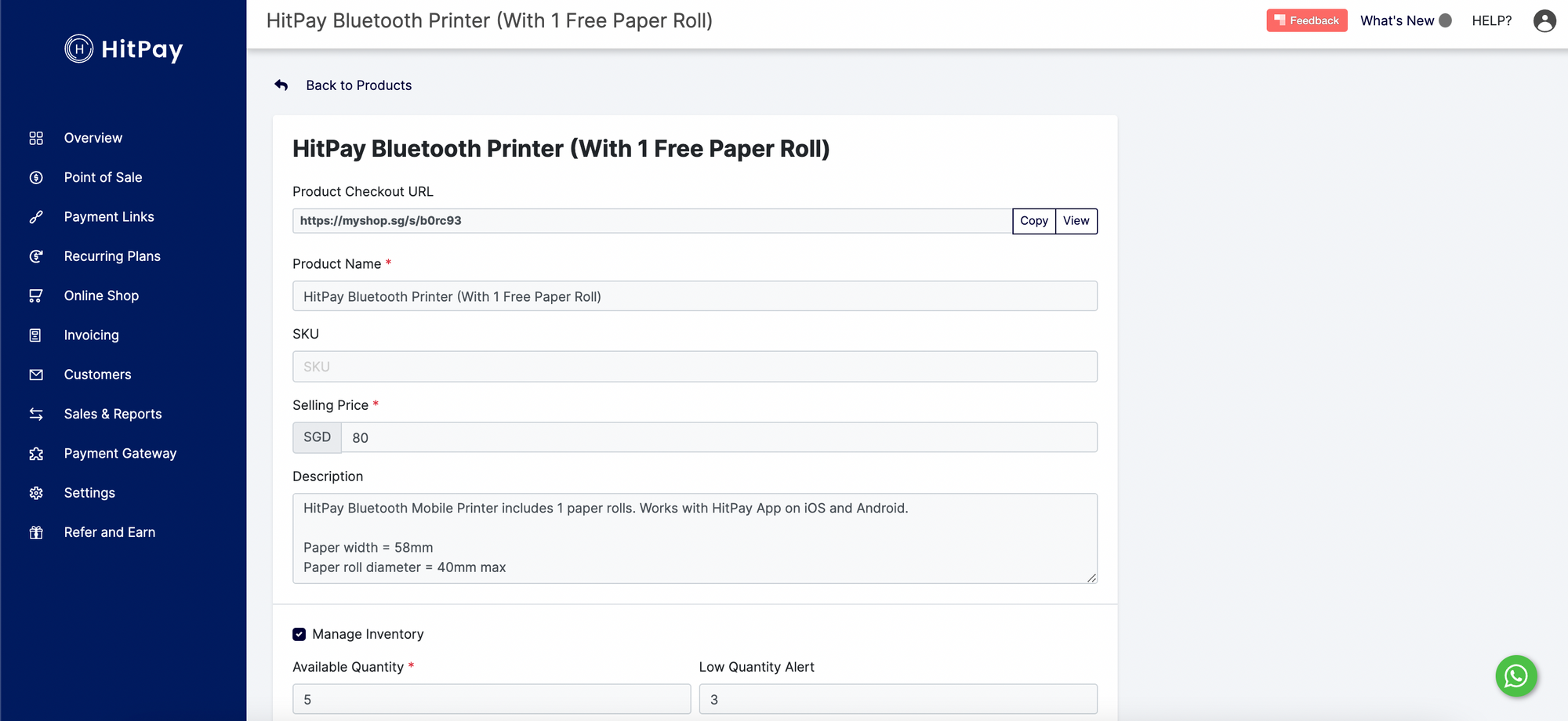The image features a user interface on a gray background, prominently displaying a white "K" alongside a white "H" inside a circle. Key sections include:

- **Overview**
- **Point of Sale**
- **Payment Links**
- **Recurring Plans**
- **Online Shop**
- **Invoicing Customers**
- **Sales and Reports**
- **Payment Gateway Settings**

There is also a "Refer and Earn" section. The interface includes a "Hit Pay" option, accompanied by a description stating "Bluetooth Printer (with one free paper roll)." Additionally, a help icon indicated by a question mark and a profile icon are visible. 

Navigation options such as "Back to Products" with an arrow pointing to the left are also included. Another "Hit Pay" option, again noted as "Bluetooth Printer (with one free paper roll)," is present. 

For product management, a "Product Checkout URL" is displayed with actionable options like "Copy" and "View" beside two gray rectangles. The "Product Name" field is marked with a red asterisk indicating it is mandatory. A SKU field is present, with a box for entering the selling price, listed as 80. 

There is also a description box for additional information and a "Manage Inventory" checkbox that is checked. The interface displays "Available Quantity" as 5 and a "Low Quantity Alert" set to 30.